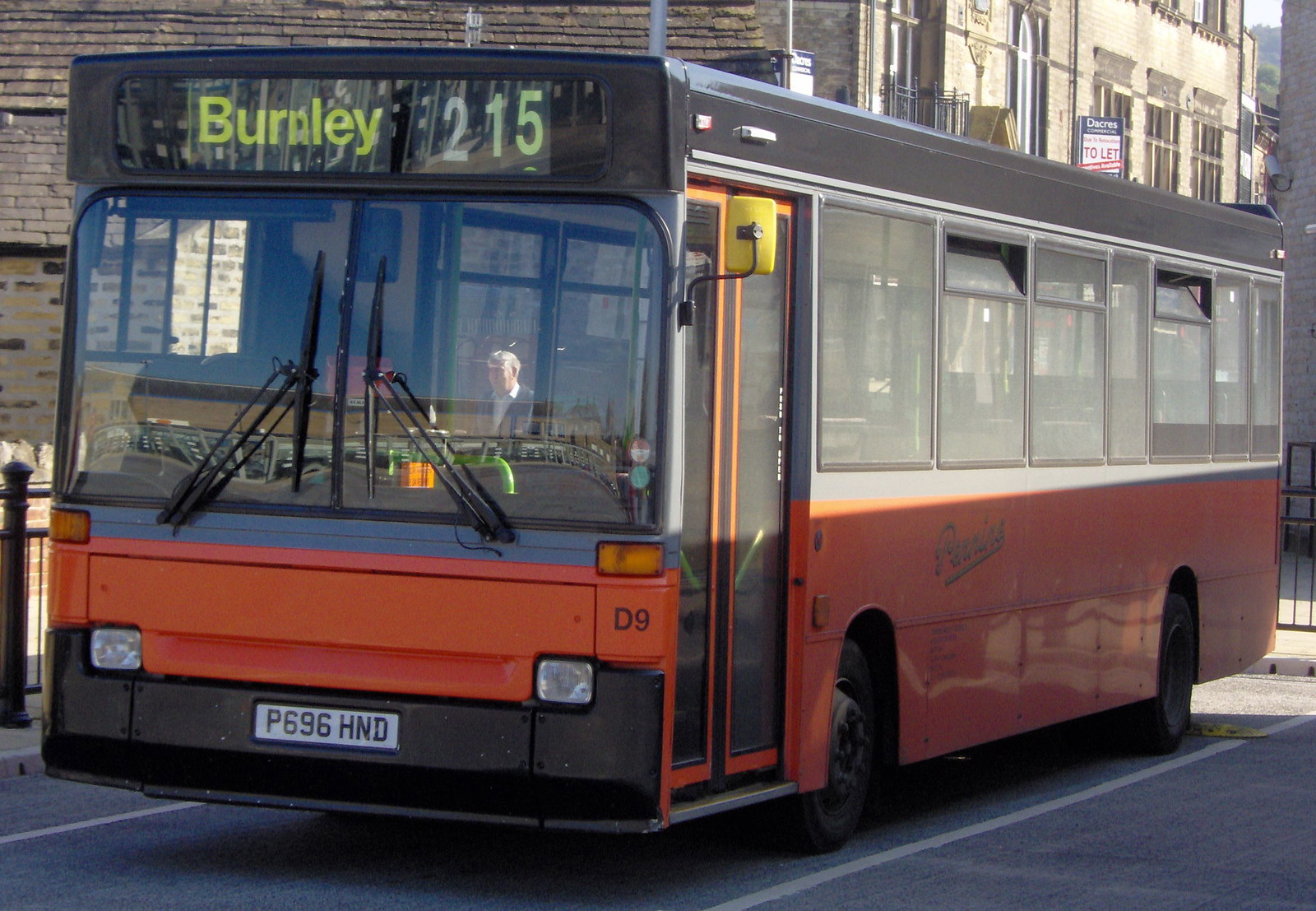The photograph captures a city bus prominently positioned in the center of the image, occupying most of the frame. This large, blocky, and square-shaped bus features a striking color scheme with a black top and a vivid orange lower section. The LED sign at the front of the bus reads "Burnley 215" in off-green text. The front of the bus also displays a white license plate with black text, reading "P696 HND," alongside additional markings like "D9" on the lower right corner.

The bus appears to be parked, not in motion, situated between two white lines on the street, suggesting it is in a designated bus parking spot. The windshield is equipped with centrally attached black wipers, and the windows along the side reveal no passengers or driver. One observer notes seeing a person appearing through the windshield and side windows, actually walking on the sidewalk adjacent to the bus.

In the background, various buildings are visible, including brick structures in brown and black, and a prominent cream-colored brick building. There's also a sign reading "To Let," indicating nearby apartment buildings. The scene is set outdoors with visible asphalt and shadows cast by the bus, hinting at the sunny condition. Additionally, some black fencing appears intermittently at the edges of the frame, partially obscured by the bus itself.